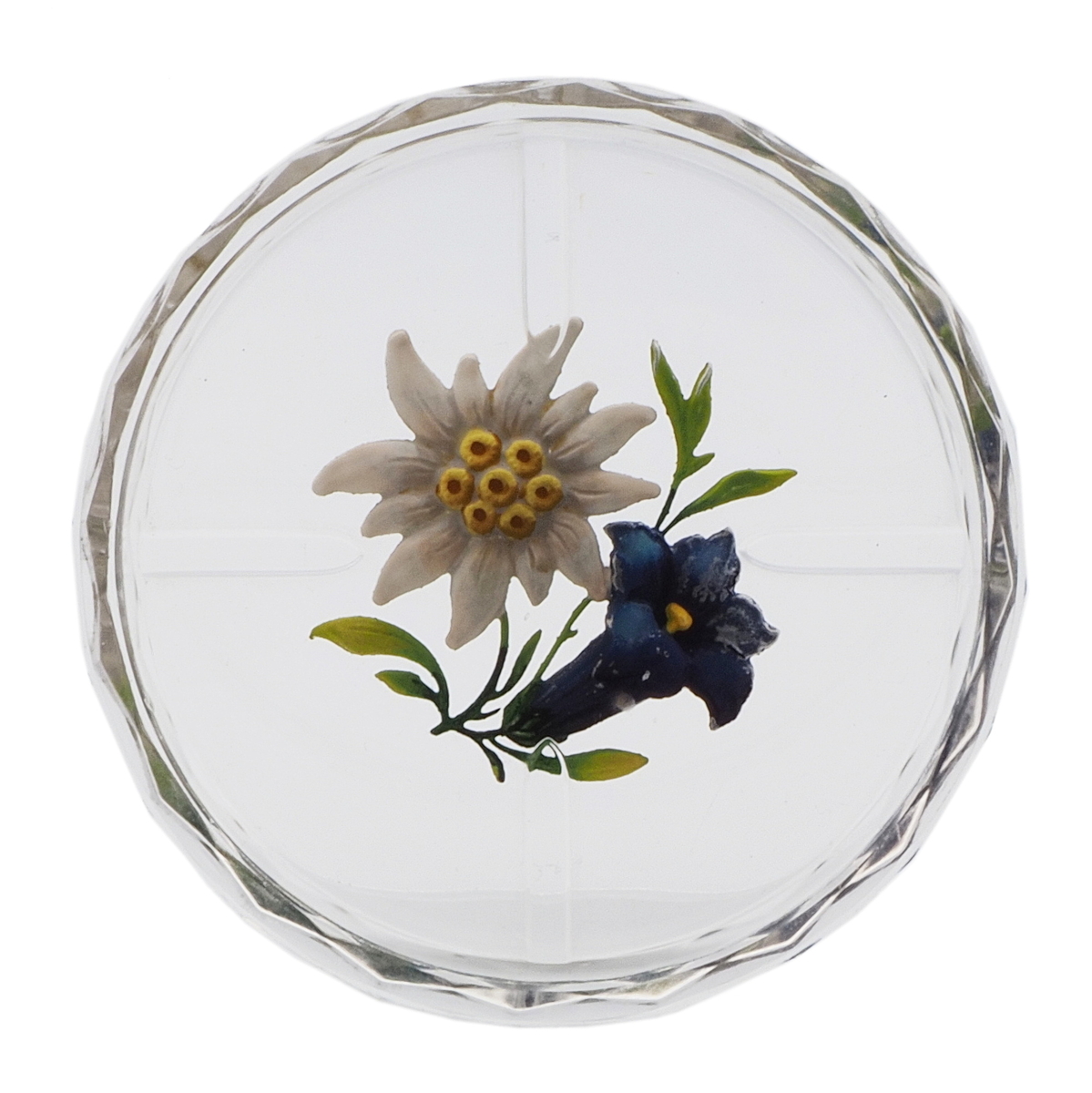The decorative object in the image appears to be either a plate, a wall hanging, or some form of porcelain or crystal ware, viewed from a top-down perspective. The object is circular with a wavy, undulating rim, suggesting the intricate edge of a crystal vase or the artistic design of a painted plate. The rim is adorned with four small indentations or raised elements positioned at the equivalent of 12, 3, 6, and 9 o'clock. The center features two floral designs: a large white blossom with yellow stamens and a tall blue flower, possibly a morning glory, accompanied by a smaller yellow element. These flowers are connected by a shared vine with five green leaves, highlighting their relation despite their different colors. The background of the object is primarily white, surrounded by a grayish, ornate border that resembles netting. The overall design conveys a floral, spring-like theme, making it a suitable decorative piece for hanging or display rather than practical use.